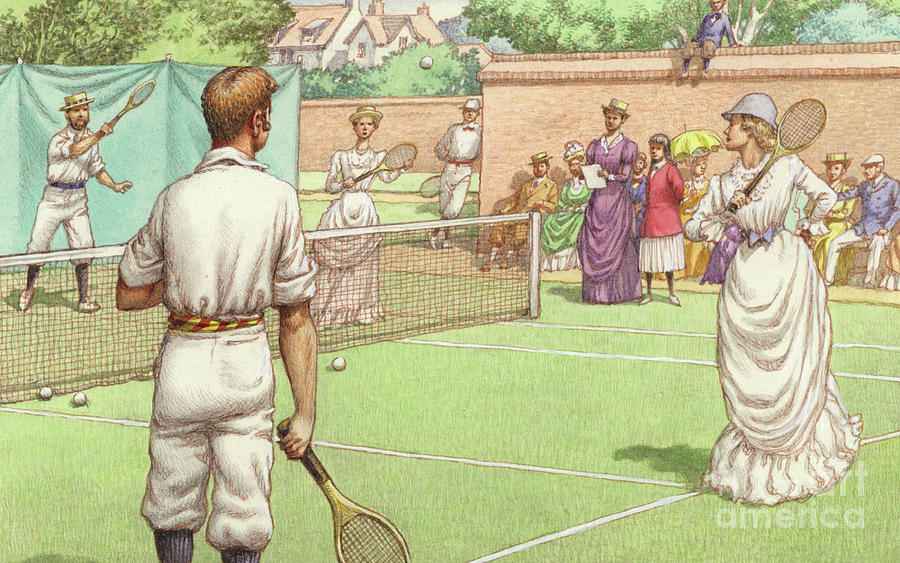This is a detailed illustration of a Victorian-era mixed-gender tennis match set in the 1800s. The horizontal rectangular drawing features a light pink tennis court divided by a net. On the near side of the net, a man and a woman are positioned to play: the woman, dressed in a full-length, white dress, is holding it up to run, and she has a tennis racket in her other hand. She also wears a hat. The man, seen from the back, is clad in white pantaloons and a collared shirt tucked into his belt, holding a tennis racket. The opposing couple on the far side of the net is similarly dressed. Surrounding the court is a scene of spectators dressed in Victorian attire, including women in colorful dresses – one with an umbrella, a woman judge in a purple dress with a paper, and men in fancy suits. Behind them, a brick wall extends along the background, with some people sitting on it and others leaning against it to get a better view, including a boy. Beyond the wall, trees and large houses complete the idyllic, historical setting.